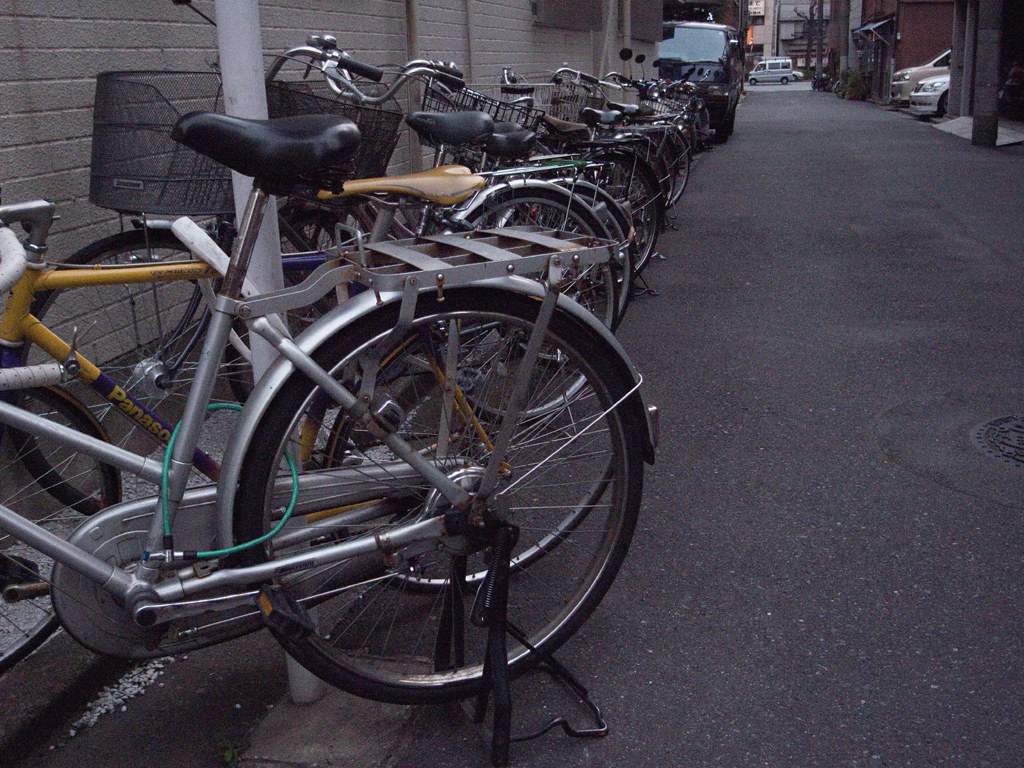This horizontal rectangular photograph vividly captures an alley lined with various parked bicycles on the left side against a gray brick building. The alley, paved in clean black asphalt, runs from the foreground to a main street in the background, where a white van is visible driving past a parked car. On the right side of the alley, one can spot parked cars behind a fence, a telephone pole, and a parking lot with brick buildings and a garage further down. In addition, a black van is parked at the far end of the alley on a perpendicular street.

The bicycles, amounting to approximately 10 or 11, are parked in a neat row, one next to another, featuring diverse colors like silver, yellow, blue, and green, with most seats being black and a few brown. Some bicycles boast additional features like baskets, rearview mirrors, and bells, while others are secured with chains or locks. Notably, a yellow bicycle with a blue stripe has partially obscured yellow text, possibly spelling "Panasonic." The scene also includes vertical white poles along the wall and a shrub near the awning of an adjacent building, hinting at a blend of urban functionality and subtle greenery. The photograph, taken during daytime, offers a meticulous glimpse into this tranquil alleyway, showcasing a typical urban setting where bicycles are prominently used for commuting.